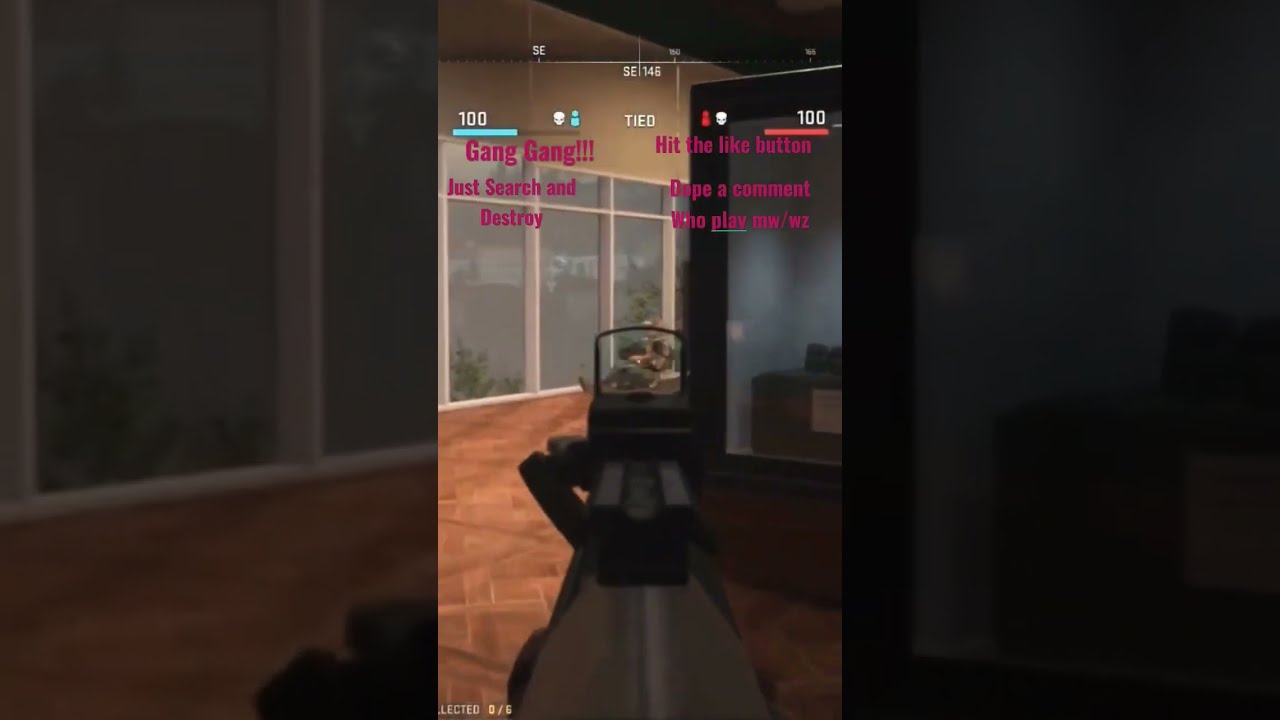This is a screenshot from a TikTok video featuring a 3D shooter video game. The image focuses on a narrow vertical frame, likely derived from a mobile game, with blurred and zoomed-in side borders to fill the space. The primary scene displays a first-person view through the scope of a gray sniper rifle or magnifying gun sight, aimed at a target sitting in a lounge chair. The setting appears to be an interior space, possibly an apartment or hotel room, with wood floors, wide ceilings, and glass walls showing trees outside. A HUD at the top features directional indicators and mirrored scores, both displaying 100 with blue and red lines. An overlay of pink text reads, "gang gang just search and destroy. Hit the Like button. Drop a comment. Who play MW/WZ?"